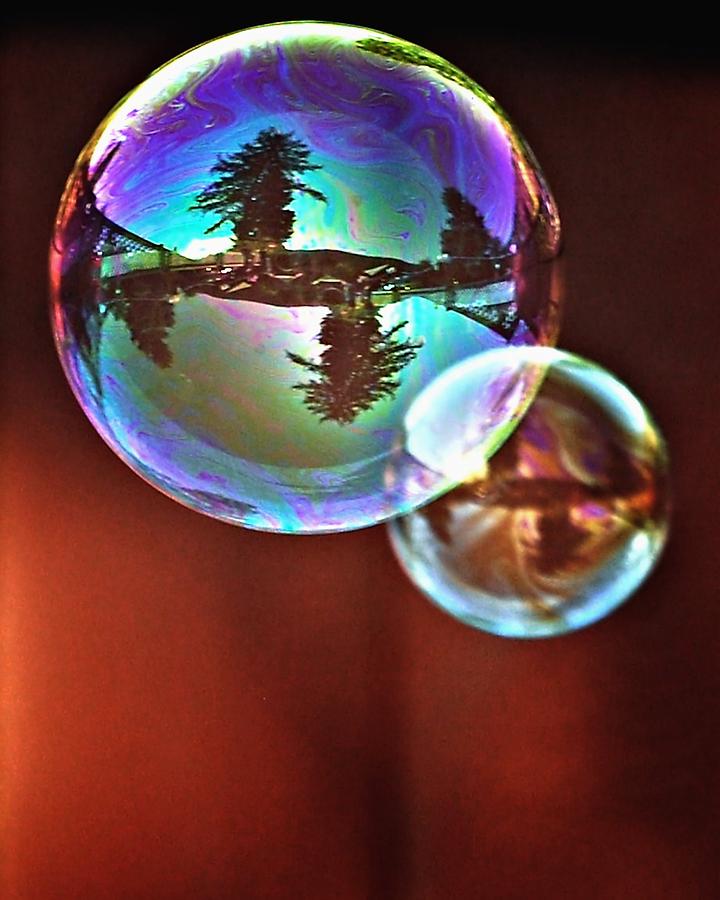The image showcases two intricately detailed soap bubbles against a burnt sepia brownish-orange background that darkens to almost black towards the top. The larger bubble, positioned slightly to the left, prominently displays an iridescent array of purples, blues, greens, and oily textures. It captures the reflection of an outdoor environment, including a large tree, situated just left of the center, another evergreen tree to the right, and a possible fence and house with the sky visible behind them. This reflection is mirrored upside down on the bottom half of the bubble, enhancing the illusion of depth. The smaller bubble, conjoined to the larger one at the bottom right, appears somewhat out of focus, primarily displaying indistinct swirls of brown, orange, red, blue, and yellow hues. The overall composition creates a mesmerizing effect of floating orbs encapsulating miniature landscapes within their translucent, oily surfaces.